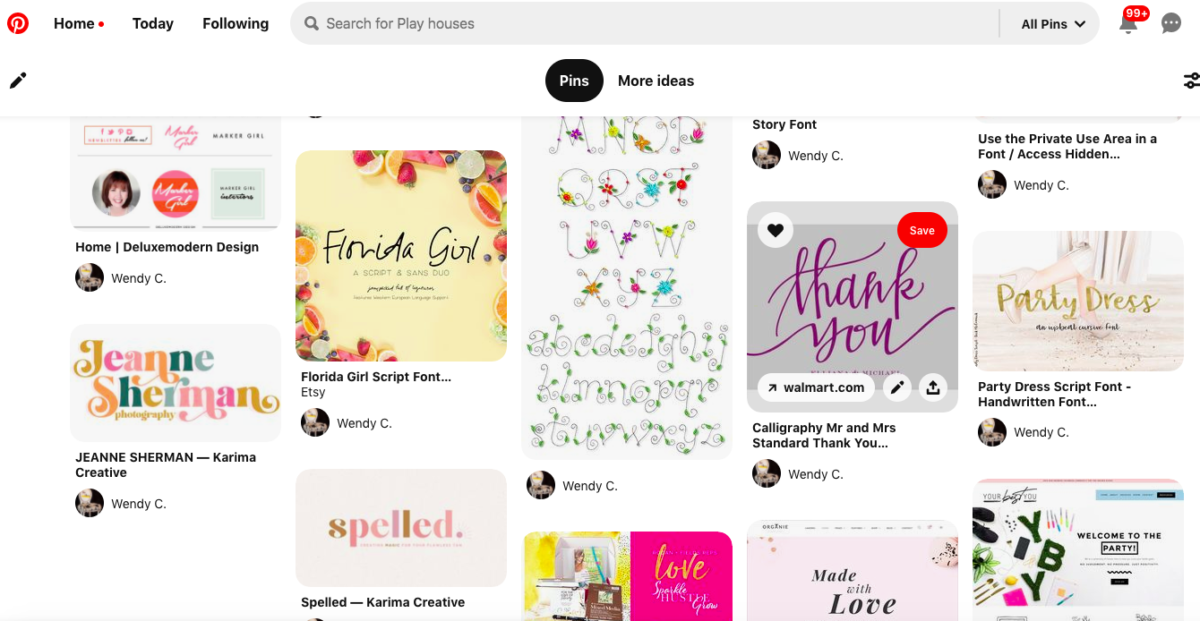**Detailed Caption for Pinterest Screenshot:**

The image is a screenshot of a Pinterest page, distinctly showcasing the interface and various content posted by a user named Wendy C. 

**Top Navigation Bar:**
- On the top left, immediately to the right of the Pinterest logo, there are three navigation links: **Home, Today,** and **Following**.
- In the center of the top bar, there is a gray oval search bar labeled **"Search for playhouses"**.
- To the right end, there is a notification bell with a red overlay indicating **"99+" new notifications. Right next to the bell is a gray speech bubble with three horizontal dots inside.

**Page Layout:**
- Below the top bar, on the far left side, a black pencil icon is visible, possibly for editing purposes.
- In the center of the same horizontal line is a black oval labeled **"Pens"** in white text. To its right, there's a link titled **"More Ideas"**.
- The far right area features filters, presumably for refining the search results.

**Content Overview:**
- The main content area displays multiple posts created by the user Wendy C. Wendy's profile picture is difficult to discern but seems predominantly black with a small white moon-like shape.
- Visible are eight posts along with snippets of two obscured posts. Each post is briefly detailed below:

  1. **Top Post:**
     - Title: **"Home Deluxe Modern Design"**
     - Visual: Screenshot possibly advertising a business related to deluxe modern design.
  2. **Second Post:**
     - Title: **"Jeanne Sherman Photography"**
     - Text Colors: Multiple vibrant shades including yellow, pink, lighter pink, orange, dark green, and muted gray-green.
  3. **Third Post:**
     - Title: **"Jeanne Sherman-Karima Creative"**
  4. **Fourth Post:**
     - Title: **"Florida Girl, script in Sans Duo"**
     - Description: Image with a pale yellow background, vibrant fruits at the top right and bottom left corners. Includes unreadable smaller text.
  5. **Fifth Post:**
     - Title: **"Spelled"**
     - Visual: Letters in mixed vibrant colors. Title reads "Spelled - Karima Creative".
  6. **Sixth Post:**
     - Content: Letters M through Z in whimsical cursive with flowers, followed by lowercase letters in cursive with leaf designs.
  7. **Seventh Post:**
     - Visual: Indistinct cartoon left, "Love" text right with yellow background on the left and pink on the right.
  8. **Eighth Post:**
     - Title: **"Story Font"**
     - Information obscured
  9. **Ninth Post:**
     - Title: **"Thank You"** in calligraphy.
     - Additional Options: Heart, a red save icon, a link to walmart.com indicated by an arrow pointing upward, pencil, and share icon.
     - Additional Text reads "Calligraphy Mr. And Mrs. Standard thank you..."
 10. **Tenth Post:**
     - Text: "Made with Love" with a predominantly pink background mimicking a splash screen.
 11. **Eleventh Post:**
     - Title: **"Use the Private Use Area in a Font / Access Hidden..."**
     - Content obscured
 12. **Twelfth Post:**
     - Title: **"Party Dress"** in a sparkly yellow cursive.
     - Description: Black illegible text, background shows a woman's legs in a gold gown and high heels, on a hardwood floor with glitter.
     - Title Text: "Party Dress Script Font - Handwritten font..."
 13. **Thirteenth Post:**
     - Visual: Another splash screen titled "Welcome to the Party" with an unreadable description.

The detailed and colorful posts reflect Wendy C.'s diverse interests ranging from typography to photography and creative design.